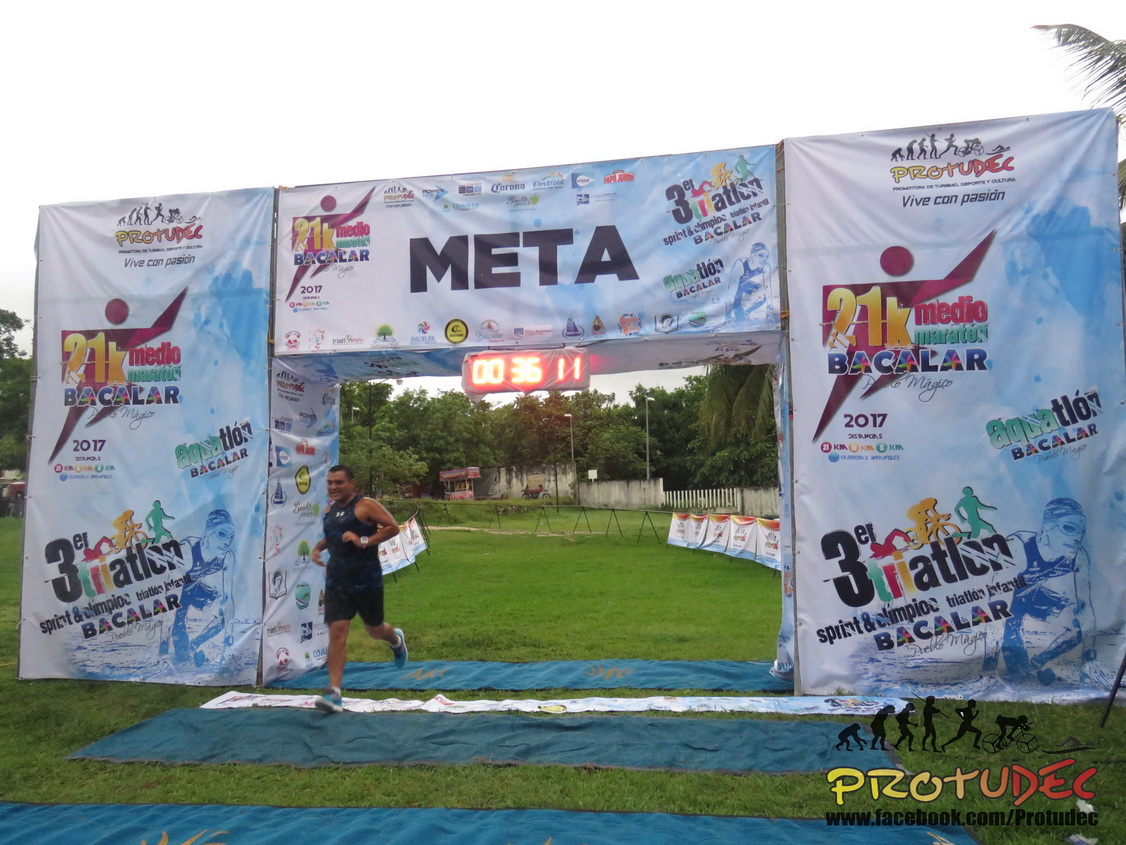This outdoor photograph captures the climactic moment of a marathon race, where a runner is crossing the finish line under a makeshift archway made of scaffolding wrapped in tarpaulin. The top of the arch prominently displays "META" in large black letters, indicating the finish line, and is adorned with various graphics and symbols, including a running man figure and logos. The signage on the tarpaulin includes "21K Marathon Bacalar 2017" in gold letters, suggesting it’s an official event, though there is no crowd visible to cheer the runner on. A digital clock above the runner shows a time of 36 minutes and 11 seconds. The runner, a man with dark skin and short black hair, is dressed in a black tank top, black shorts, and blue running shoes. Surrounding the scene, green trees and grass suggest a lush, outdoor setting. Additionally, there are various sponsor logos, including "PROTUDEC" and an image sequence of an ape evolving into a runner and then into a bicyclist on the advertising banners.